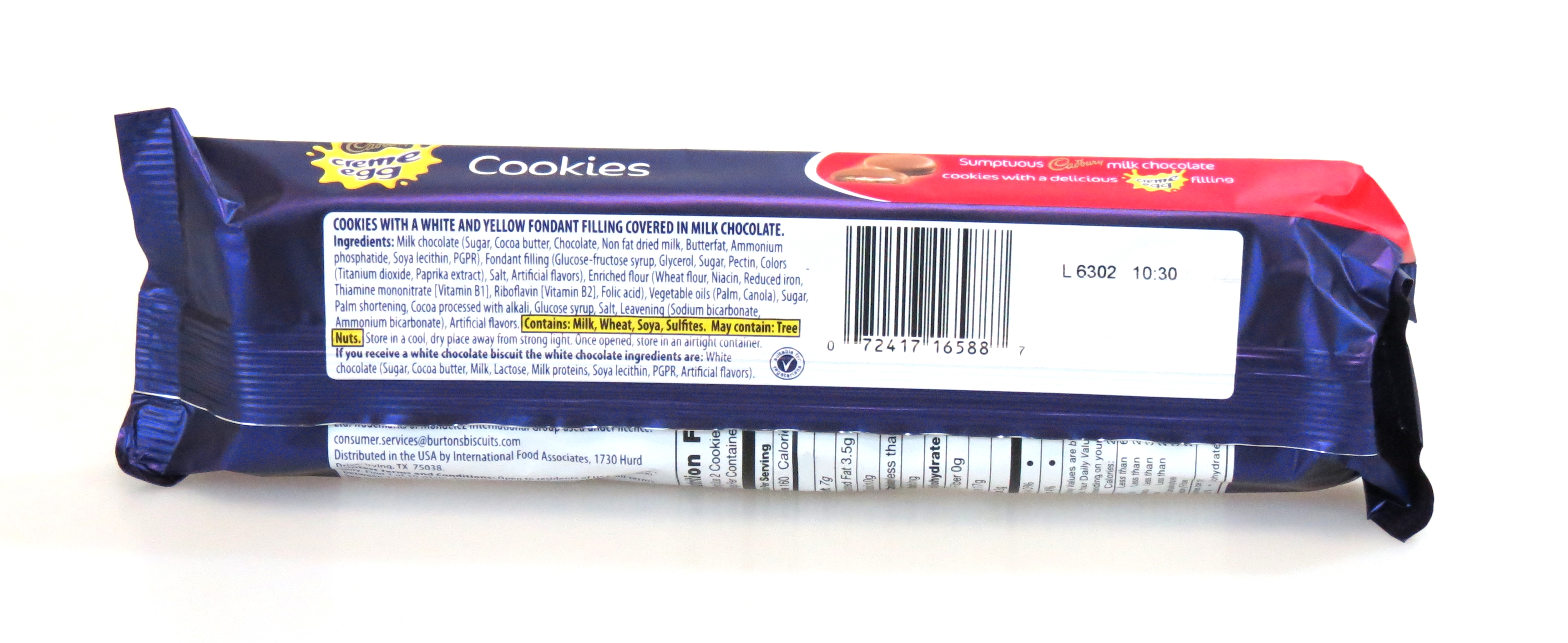This is the back side of a small, blue package of cookies. The visible portion of the package reveals the bottom segment of the label. At the top-left corner, the word "cookies" is discernible in white text, aligned towards the top-left of the package as we look at its bottom. Adjacent to this, there is a distinctive yellow splatter logo with the words "cream egg" in blue, outlined in white. While the brand name is not fully visible, the partial view of brown circles outlined in gold suggests it is likely Cadbury's signature branding.

The primary focus of this image is a white, rounded rectangular label that occupies most of the back. In blue text, it starts with the sentence "Cookies with a white and yellow fondant filling covered in milk chocolate." Below this, there is a list of ingredients that is too small to read clearly at this resolution. Some ingredients are highlighted in yellow, indicating allergens, such as milk and wheat, though parts of the list are fuzzy, leaving some items unclear.

On the right side of the package, starting from the top of the screen and extending downward, is a red section with white text, which is illegible due to resolution. Situated to the right of the main label is a barcode, followed by a code reading "L6302-1030." Further down, within the white panel, the nutritional facts are present but obscured due to the package being partially folded, rendering the specifics unreadable.